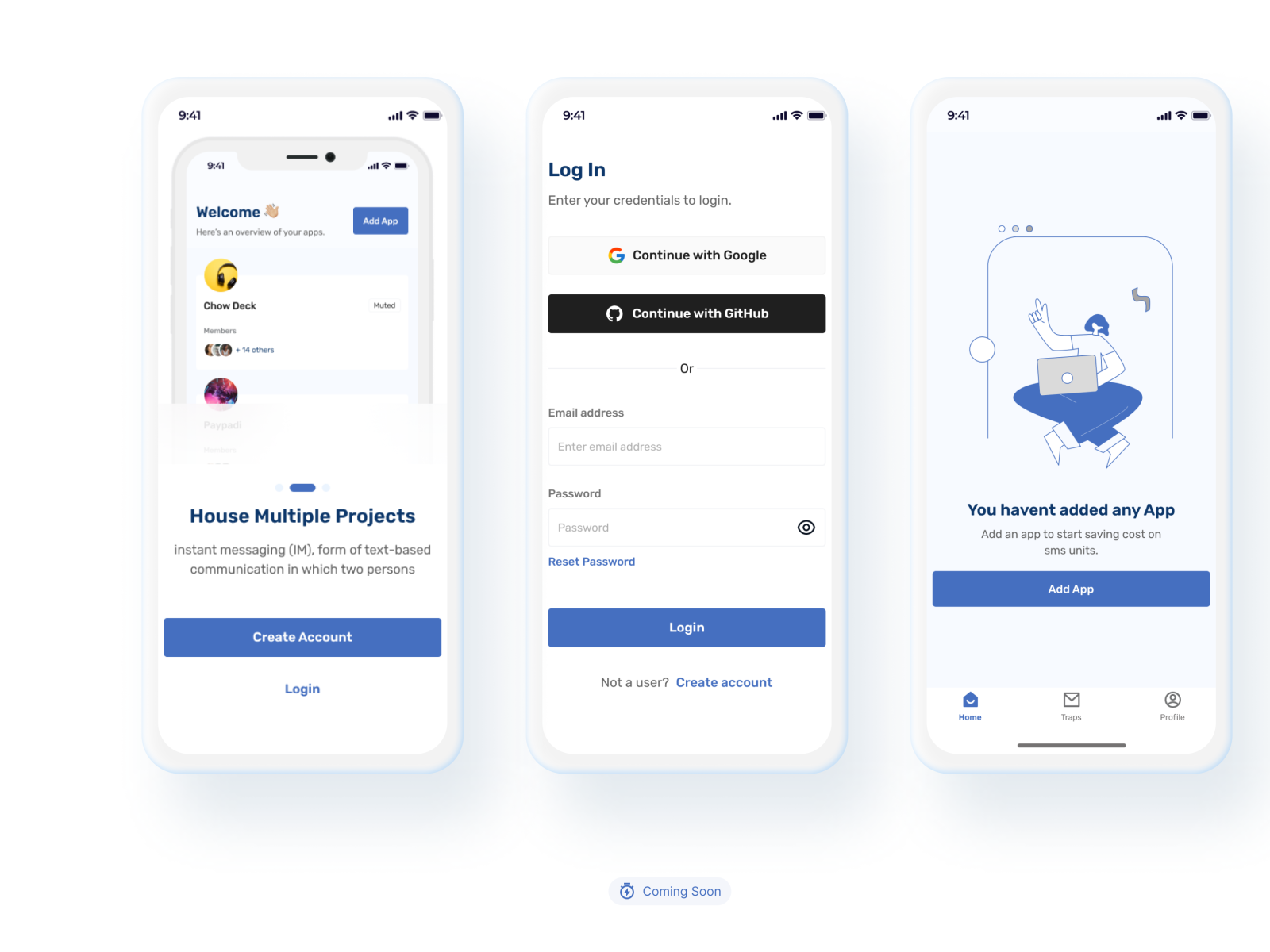The image features three screenshots, each with a gray background and the number "941" prominently displayed.

In the first screenshot, "Welcome" is written in white within a blue rectangle, followed by the text "Add App." Below this, there is information about "Shawl Deck and House" with a list of features like "multiple projects" and "instant messaging (IM)," defined as a text-based communication between two people. At the bottom, a blue rectangle contains the words "Create Account," with "Login" in blue text beneath it.

The second screenshot is a login prompt, asking users to enter their credentials. It features a gray rectangle labeled "Continue with Google" and a black rectangle labeled "Continue with GitHub," which includes an icon of a black cat in a white circle. Below this, fields are available for "Email Address" and "Password," with a link to "Reset Password" in blue. There is also a blue "Login" button. Text at the bottom reads "Not a user?" followed by a link to "Create Account" in blue.

The third screenshot shows a sketch of a person with a laptop on their lap, accompanied by the message "You haven't added any app" in blue text. It advises users to "Add an app to start saving cost on SIM units." Below this message, there is a blue rectangle labeled "Add App."

This detailed description effectively captures the design and content of the image, providing a clear and thorough understanding of its elements.